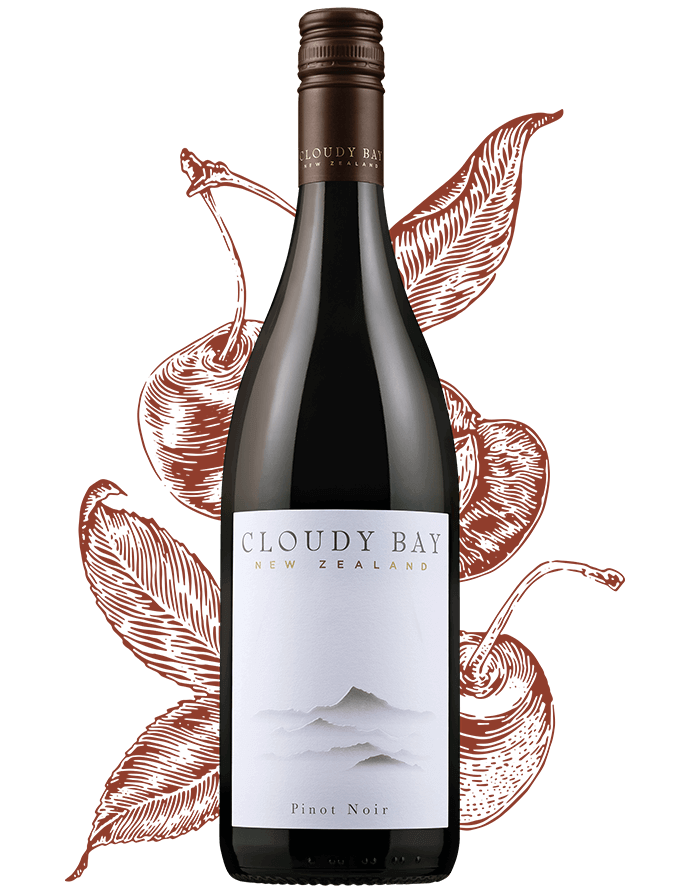This image showcases a photograph of a black wine bottle with a dark brown screw-top cap. The bottle features a white label with a detailed illustration of three to four mountains. The black lettering on the label reads "Cloudy Bay" with "New Zealand" in smaller brown print below and "Pinot Noir" further down. The background of the image incorporates a graphic design depicting two red cherries hanging from their stems among four brown leaves. This artistic presentation underscores the advertisement for Cloudy Bay, a New Zealand Pinot Noir.